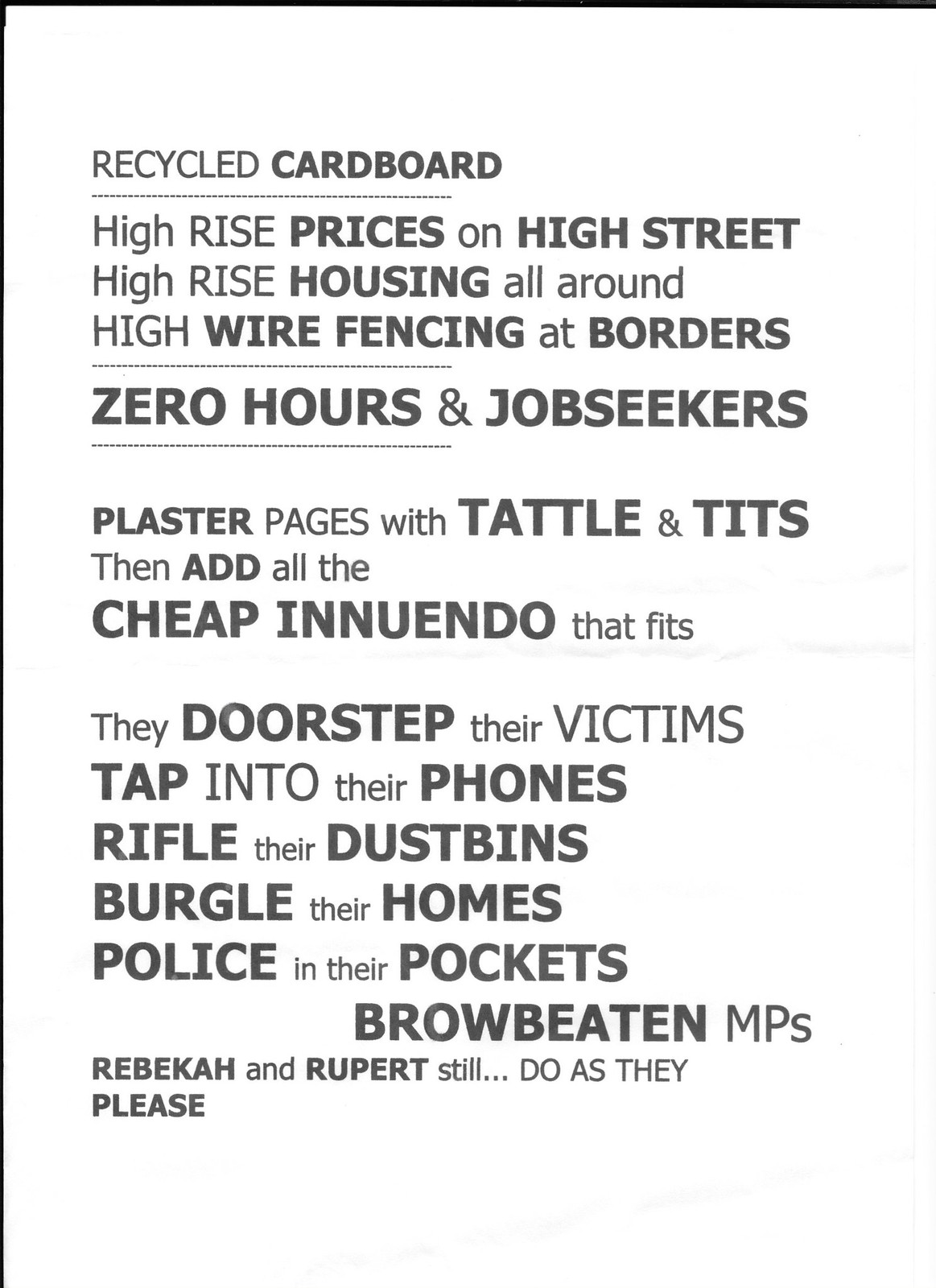The image depicts a sheet of white paper with gray text, featuring a poem that critiques societal issues in the United Kingdom. The poem highlights themes such as recycling cardboard, high prices on the high street, pervasive high-rise housing, and high wire fencing at borders. It discusses the plight of zero-hour contract workers and job seekers, and mentions the media's penchant for sensationalistic gossip ("tattle and tits") and cheap innuendo. The poem also condemns invasive practices like rifling through dustbins and burgling homes, emphasizing the power of those who "doorstep their victims," tap phones, and control the police and MPs ("browbeaten MPs"). The names Rebecca and Rupert appear, suggesting individuals who exploit these systems to their advantage. The text appears to be printed on a slightly folded paper, adding a tangible sense of urgency to its social commentary.